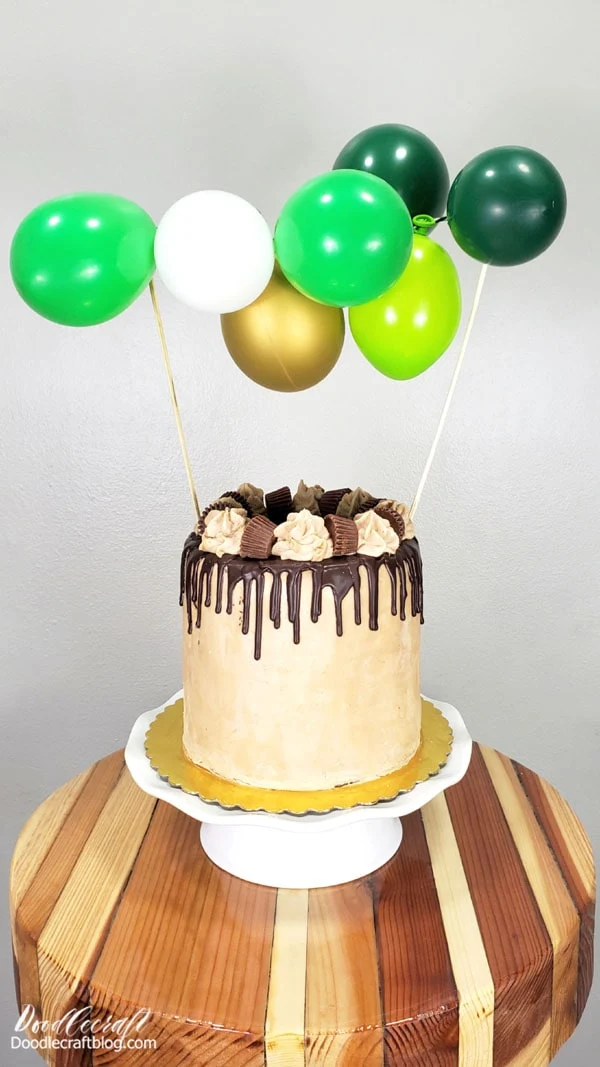The photograph, clearly a professional setup, captures a visually stunning cake intended for advertisement on doodlecraftblog.com, as indicated by the logo watermark in the bottom left corner. The background features a subdued grey, providing a neutral backdrop that accentuates the cake's details. The cake itself is elegantly displayed on a raised white platter adorned with a gold paper holder. This platter is placed on a small, round, highly glossy wooden table made up of multicolored wood slats, showcasing various shades of brown with a distinctive grain pattern.

The cake is a tall, multi-layered cylindrical confection, with an outer layer of off-white cream. It is lavishly decorated with a chocolate drizzle cascading from the top edges down the sides. At the top, the cake is garnished with an assortment of chocolate candies, including horizontally positioned peanut butter cups and white icing flowers. Two sticks rise from the center of the cake, each supporting several balloons in hues of dark green, light green, white, and gold, adding a whimsical touch to the sophisticated presentation.